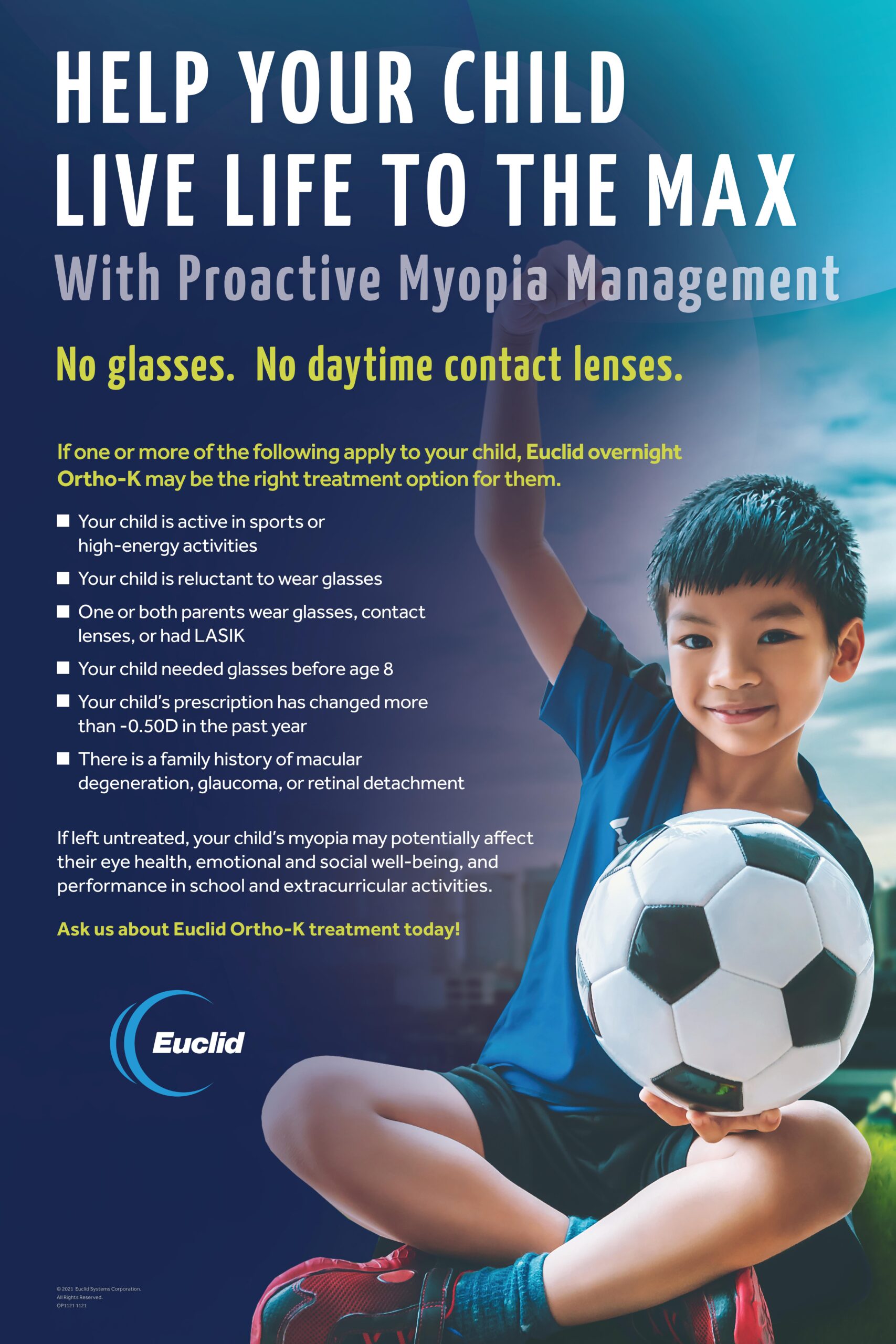The advertisement poster for Euclid's myopia management treatment features a detailed, blue gradient backdrop transitioning into a sky and green background. Prominently on the right-hand side, a photorealistic image captures a young Asian boy, approximately 10 years old, dressed in a blue polo shirt, blue shorts, greenish socks, and red and black shoes. The boy, sitting with his ankles crossed, holds a black and white checkered soccer ball while raising his right fist into the air.

At the top of the poster, in bold white lettering, the message reads: "Help your child live life to the max with proactive myopia management." Below, in yellow letters, it states: "No glasses, no daytime contact lenses." The checklist below lists factors that might make Euclid, Overnight, Ortho-K a suitable treatment option, such as if the child is active in sports, reluctant to wear glasses, or if both parents wear glasses.

Additional criteria include parents having contact lenses or previous Lasik surgeries, the child needing glasses before age eight, a prescription change exceeding minus 0.5 diopters in the past year, and a family history of macular degeneration, glaucoma, or retinal detachment.

At the bottom left corner, the Euclid logo is displayed alongside a trademarked informational segment, emphasizing the potential positive impact of treating myopia on children's eye health, emotional and social well-being, and performance in school and extracurricular activities.